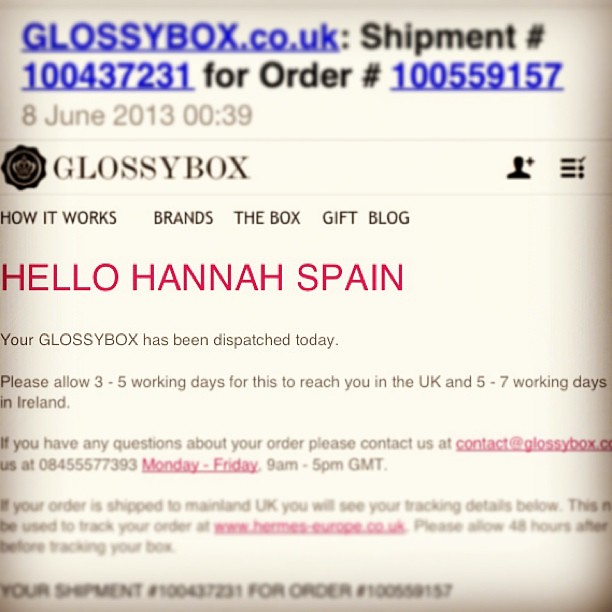The image is a screenshot of an email from Glossybox.co.uk concerning an order. At the top, a blue header reads "Glossybox.co.uk" followed by "Shipment number 100437231" and "Order number 100559157", dated "8 June 2013, 00:39". Beneath this, a black Glossybox logo is displayed next to a submenu with options: "How it Works," "Brands," "The Box," "Gift," and "Blog". The message prominently addresses the recipient with "Hello, Hannah Spain" in large red text. The email details that the Glossybox has been dispatched, advising a delivery time of 3-5 working days for the UK and 5-7 working days for Ireland. It also provides contact information for further inquiries at "contact@glossybox.com." The image features a tilt-shift blur, focusing on the "Hello, Hannah Spain" greeting while the surrounding details, including shipment and order numbers, are slightly blurred.